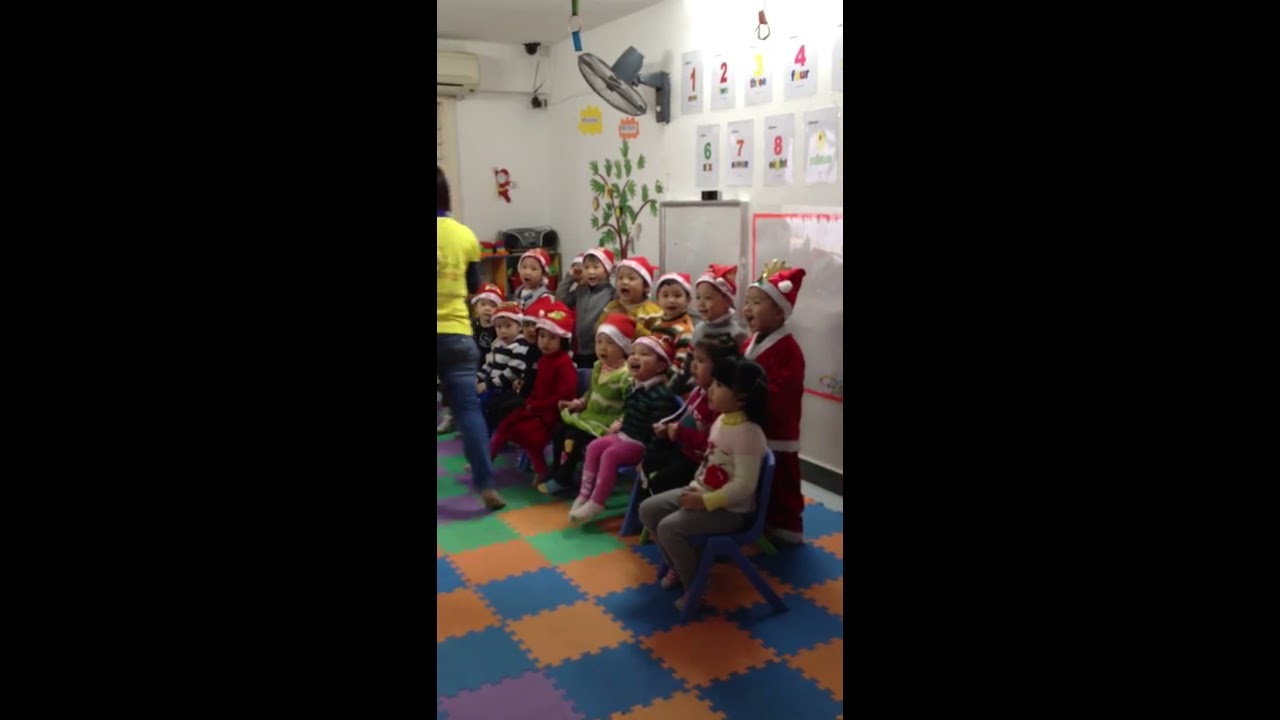In the photograph, a group of young children, likely between preschool and kindergarten age, are captured in a classroom setting performing a winter concert. Most of the children, who appear to be of Asian descent, are wearing festive red Santa hats with white trimming and pom-poms. They are arranged in two rows: a seated row in front and a standing row behind. The classroom features a checkered foam floor with interlocking pieces in orange, green, blue, and some purple squares designed like puzzle pieces. On the wall behind the children, various educational items are visible, including whiteboards, colorful numbered papers, and a painted tree. A table fan attached to the wall and an air conditioner in the top left corner contribute to the room's atmosphere. To the left of the image, partially visible, stands an adult in blue jeans and a light-colored shirt, facing away from the camera. Despite the black borders framing the image, the children's joyful expressions and their synchronized singing highlight the festive and cheerful mood of this classroom performance.